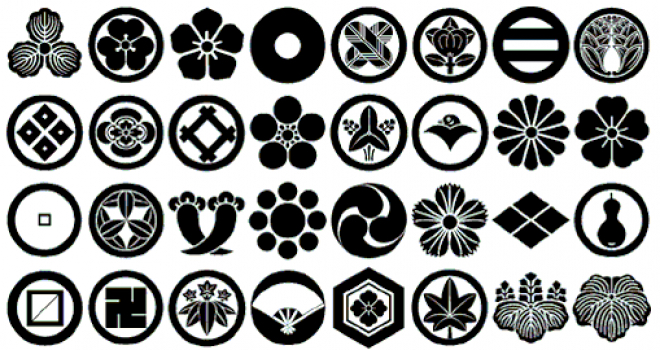This image features 32 black and white icons arranged in a grid of 8 across and 4 rows. A majority of these icons are circular, though there are 9 exceptions without rotational symmetry. Focusing on the bottom row from left to right: the first icon is a black circle containing a hollow black square. The second icon is a black circle with a black swastika in the center, a symbol originally of religious significance in Jainism but later appropriated by the Nazi party. The third icon is a black circle featuring an inverted black leaf with three smaller leaves positioned upright atop it. The fourth icon is a black circle centered with a white handheld fan. The image's stark black and white palette highlights these symbolic forms.